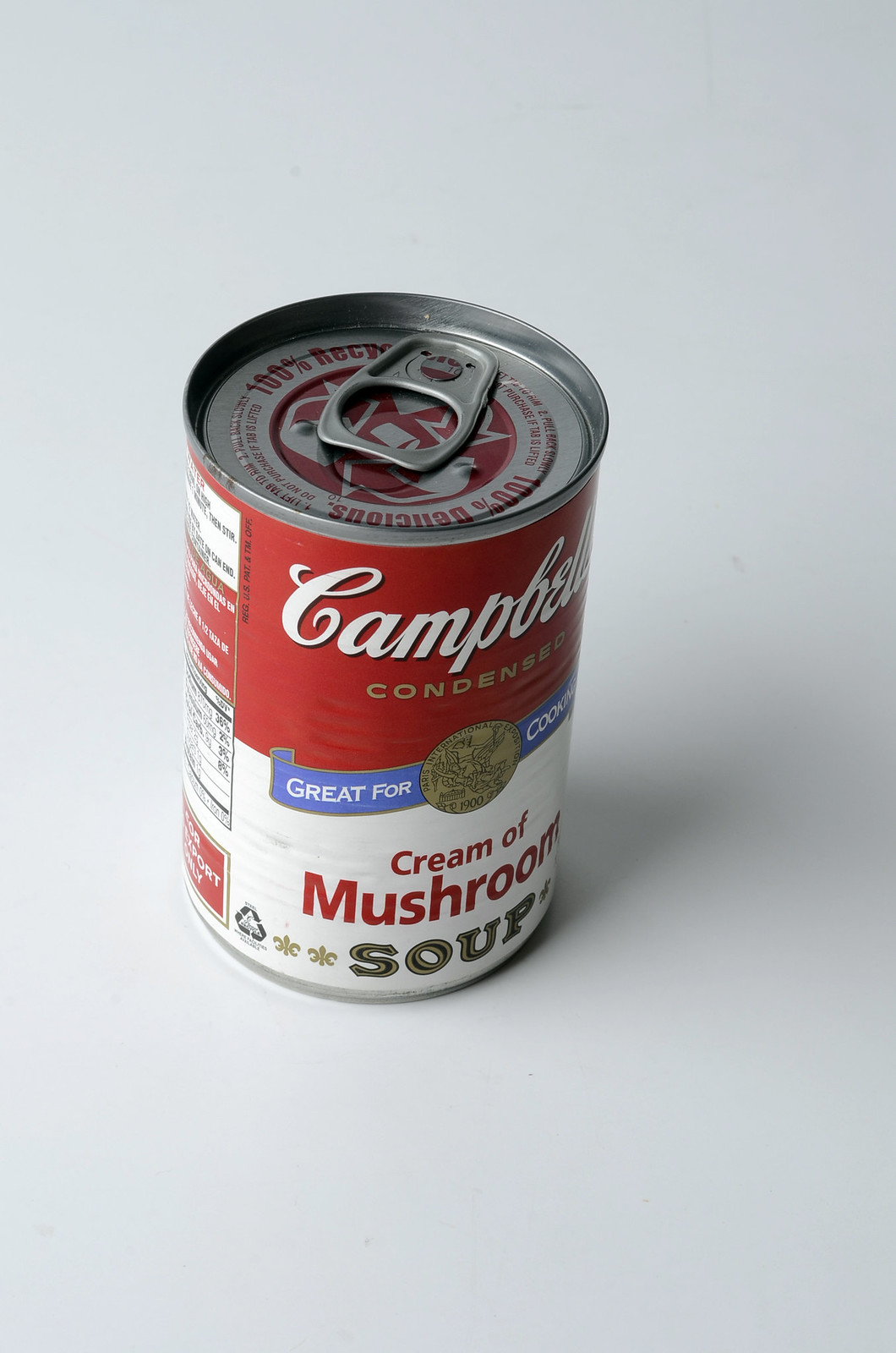The photograph features an unopened can of Campbell's Cream of Mushroom Soup, placed against a white background that gradates into gray towards the top. The can includes a pull top for easy opening. The upper section of the can showcases the familiar red Campbell's branding, adorned with a blue ribbon and a gold medallion in the center. Below this, the label transitions to white, with "Cream of Mushroom" written in bold red letters and "Soup" displayed in a combination of gold and silver lettering. Partially visible text indicates "Great for Cooking" wrapped around the label. To the left side of the image, the nutritional information and ingredient list are angled slightly out of view. Additionally, there's a recycling symbol marked by a triangle, suggesting the can is recyclable.